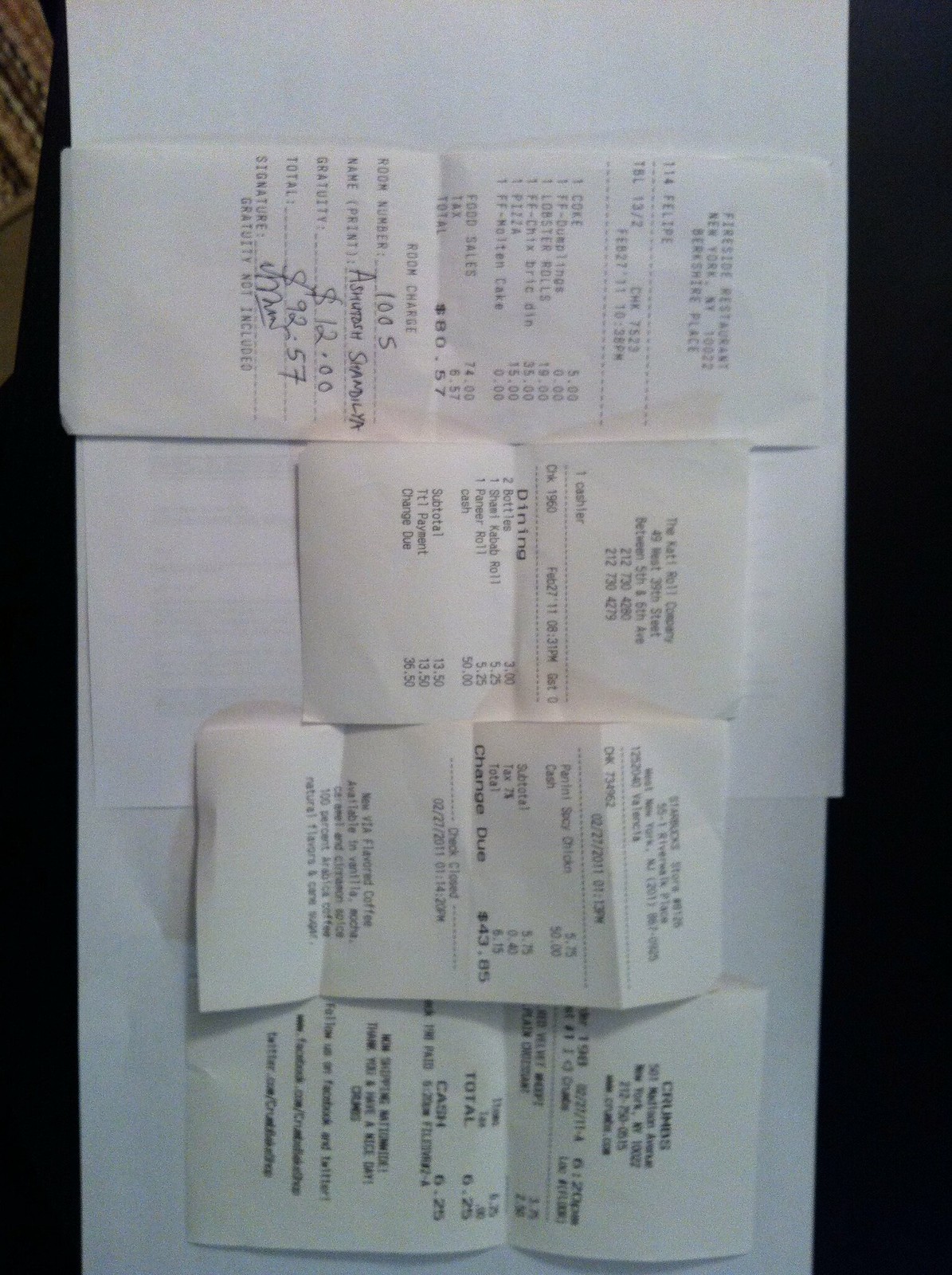This photograph captures a series of horizontally arranged receipts placed on top of a white sheet of paper, which itself rests on a black background. The image is oriented sideways, making the receipts appear vertical from top to bottom. The topmost receipt is from Fireside Restaurant located in New York, New York, 10022, Bereshire Place, and details several food items totaling $80.57. Beneath this is another receipt labeled "Room Charge." The following receipt is from the Caddy Roll Company at 49 West 39th Street, between 5th and 6th Avenue, showing food items totaling $36.50. Next is a receipt from a Starbucks Store for items totaling $6.15. The final receipt is from Crumbs at 501 Madison Avenue, listing various food items totaling $6.25. The receipts are white with black text, some featuring handwritten notes, including amounts like $12.00 and $9.25. The paper they rest on shows faint printing visible through its folds, hinting they might serve a demonstrative purpose. A slight glimpse of a wooden surface beneath the paper is visible, partly obscured by shadows, adding to the overall complexity of the layered arrangement.